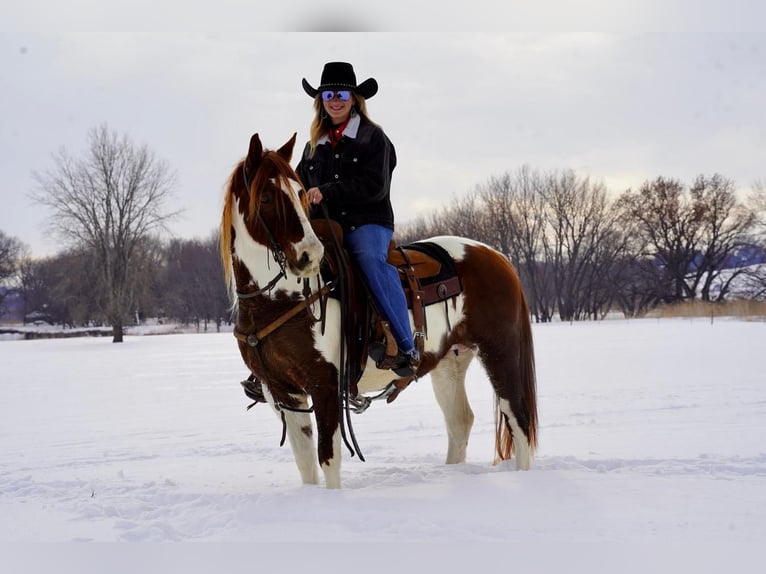A striking portrait captures a woman happily sitting on a brown and white spotted horse amidst a deep, snowy landscape with bare trees in the background. The woman's dirty blonde hair peeks out from beneath her black cowboy hat, and she wears reflective sunglasses, a black long-sleeve jacket with a white collar over a red undershirt, and blue jeans. The horse's blonde mane and tail contrast beautifully with its coat, which resembles a cow pattern with white legs and large brown splotches. The snow-draped field, marked only by their tracks, creates a stark, monochromatic backdrop that emphasizes the serene and wintry setting. The woman is smiling warmly at the camera, her hands resting on the brown saddle, looking content and at ease.